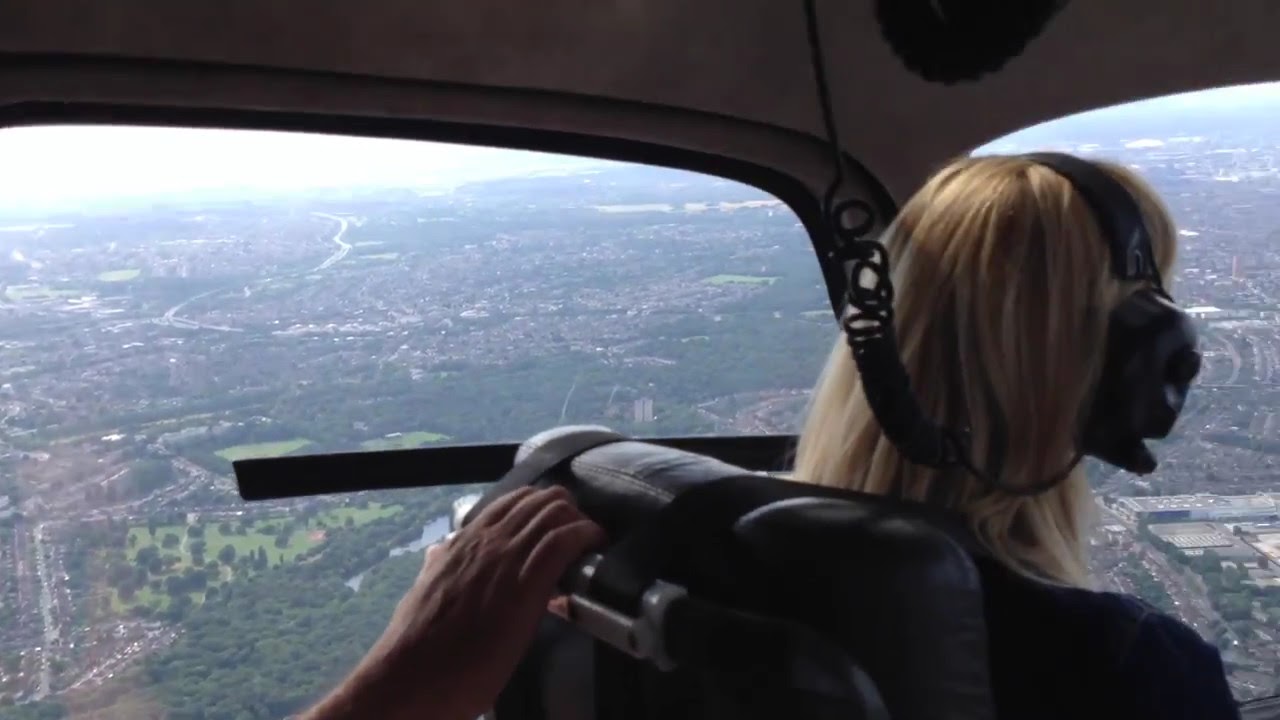This is a daytime color photograph taken from inside the cockpit of a helicopter in landscape orientation. The image captures a detailed aerial view of a slightly foggy residential cityscape below, featuring a landscape with numerous trees, houses, winding roads, and a river. The aerial perspective reveals parks and urban development within the city area.

Inside the helicopter, we are positioned behind the pilot on the left-hand side. A woman with long blonde hair, seated in a gray cushioned chair with shoulder harness straps, is visible in the right-hand side of the image. She is wearing a black top and an over-the-ear black headset typically used by pilots and passengers. The back of her head and her seat are prominent in the foreground. Additionally, a tanned hand extends from the bottom left, gripping the back of her chair. Expansive windows offer views both front and side, accentuating the vast landscape and urban sprawl beneath. The ceiling of the helicopter's cockpit is partially visible overhead.